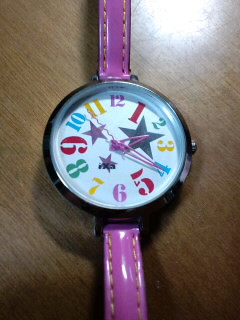The image features an analog watch lying on a light brownish, wood-like table. The watch bands, located at the top and right of the image, are a vivid bright pink leather, with a thin wrist strap that suggests it may be designed for a child. The watch face is completely white, encased in what appears to be a black plastic or metal frame. The numbers on the face are large and whimsically colored, with standout digits like a giant pink 1, a yellow 3, a red 5, a pinkish-red 9, and a yellow 11. Additionally, the watch shows an assortment of other colors such as green, tan, and blue for the numbers. The hands of the watch are also in pink, with the second hand characterized by a squiggly design, while the hour and minute hands are pointy. Surrounding the numbers, there are four stars: one near 1, 2, and 3, one just above the 7, one under the 10, and one more above the 7, accompanied by black lettering spelling out "VXA." The setup of the photo suggests the presence of a circular flash on the upper right, adding a reflective white highlight to the scene.